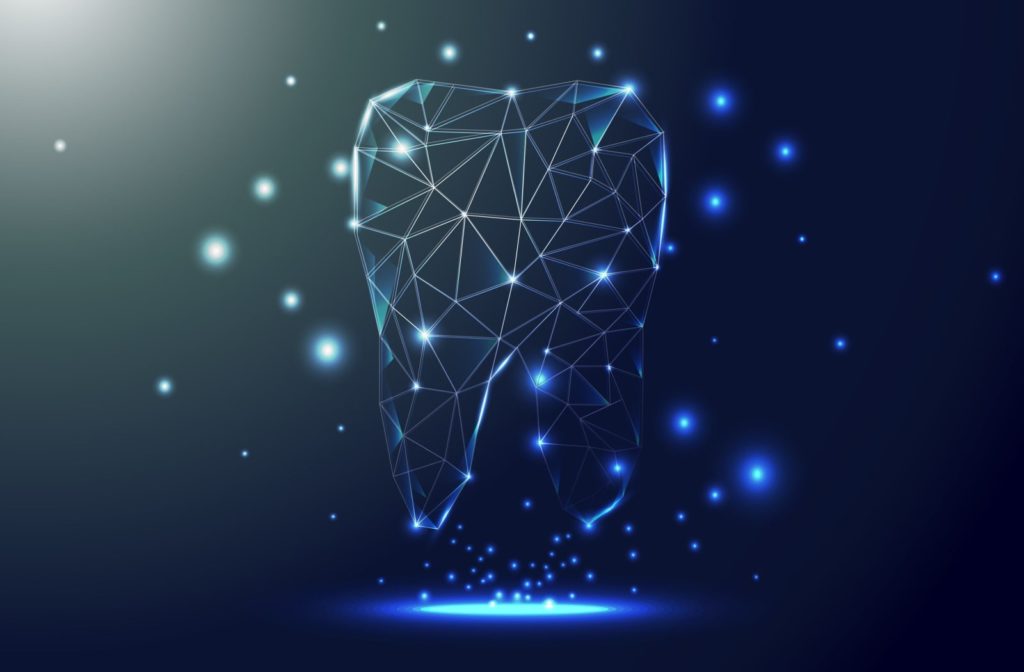This digital illustration features a large, prism-like molar tooth composed of interlocking triangles, creating a semi-transparent, faceted appearance. The tooth is centrally positioned, appearing to levitate against a dark blue and black background, which transitions from a darker hue on the bottom right to a lighter shade in the upper left corner. Surrounding the tooth are various lights: the right side is dotted with darker blues, while whiter lights illuminate the left, giving the impression of stars in a cosmic scene. Numerous light speckles appear to fall from the tooth's roots down to a bright light blue circle on the ground directly below it, suggesting a spotlight effect that fades into the dark backdrop. The tooth itself sparkles with lights of light and dark blue, highlighting the intricate design and 3D modeling technique used in the artwork.